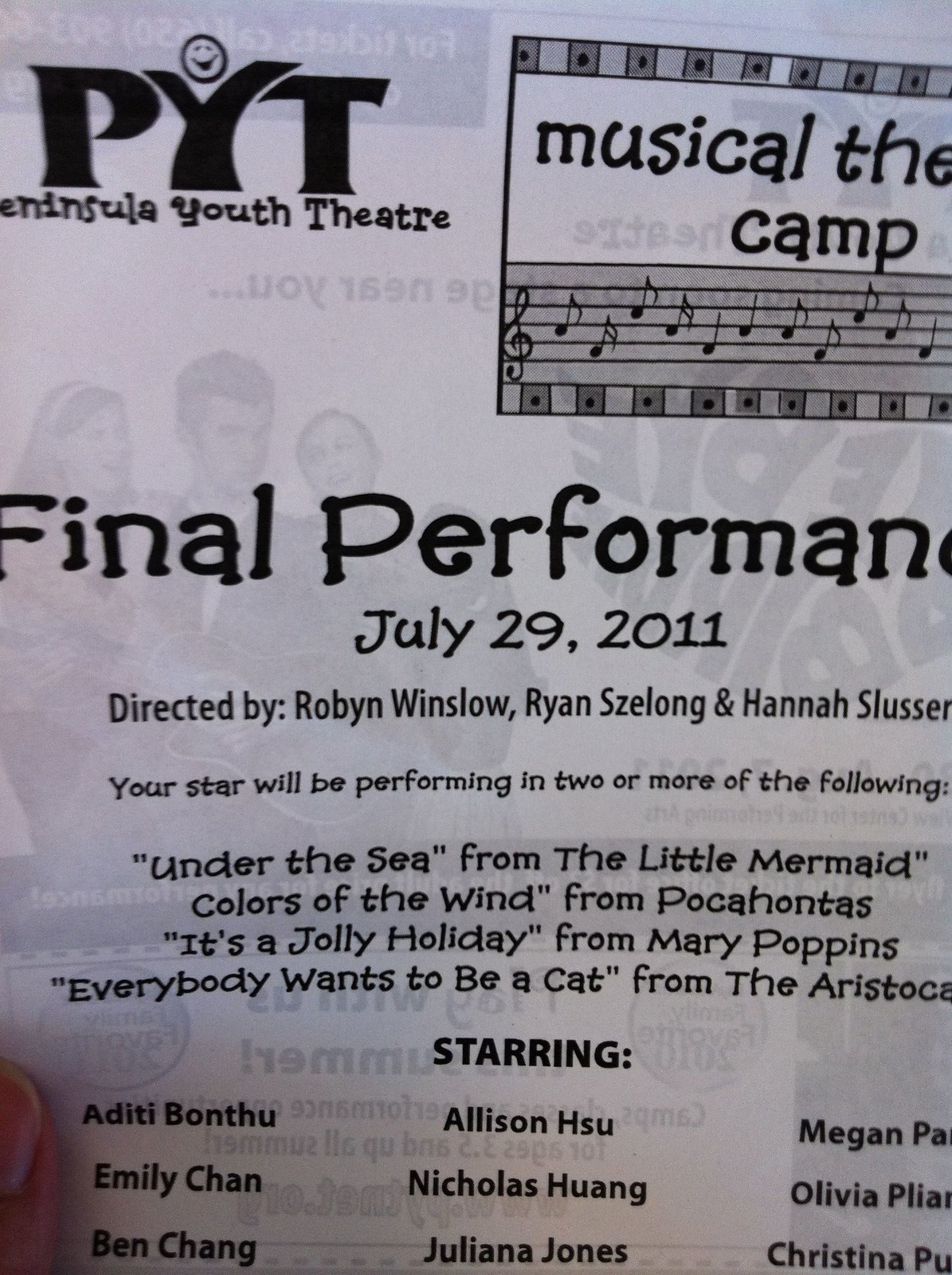The image depicts a section of a program from the Peninsula Youth Theater, printed on white paper with black text. In the upper left corner, there is the PYT Peninsula Youth Theater logo, accompanied by a smiley face above it. To the right of the logo is a box containing musical notes and the text "Musical Camp." At the lower left of the image, a peach-colored finger partially holds down the paper. The title below the box reads "Final Performance, July 29, 2011," directed by Robin Winslow, Ryan Zulong, and Hannah Slusser. In the background, a faded image of performers can be seen. Below the directors' names, the text indicates that the performance features songs such as "Under the Sea" from The Little Mermaid, "Colors of the Wind" from Pocahontas, "It's a Jolly Holiday" from Mary Poppins, and "Everybody Wants to Be a Cat" from The Aristocats. The list of starring performers includes names like Atita Banthu, Emily Chan, Ben Chang, Allison Hsu, Nicholas Hwang, Juliana Jones, Megan Pa, Olivia Plia, and Christina Pu, though some names are partially cut off.